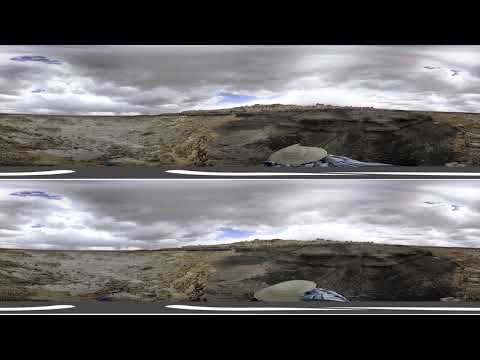The image is a split, panoramic-style photo showing a rural canyon environment, taken with a fisheye lens. The top and bottom halves are nearly identical, perhaps captured seconds apart. It depicts a cloudy sky with a few blue patches breaking through and a vast, open field or rocky desert landscape below. There is a large, dark rock formation on the right, which might suggest a history of mining, given the cutaway appearance and the contrast with the lighter-colored rocks nearby. The scene, likely from a 360-degree or panoramic photograph, is devoid of people or text, though a faint cream-colored oval and a bluish-gray object can be spotted in the lower third of the image. The photographer, wearing a hat, appears in the center, taking a selfie in this potentially Grand Canyon-like or similar canyon area.